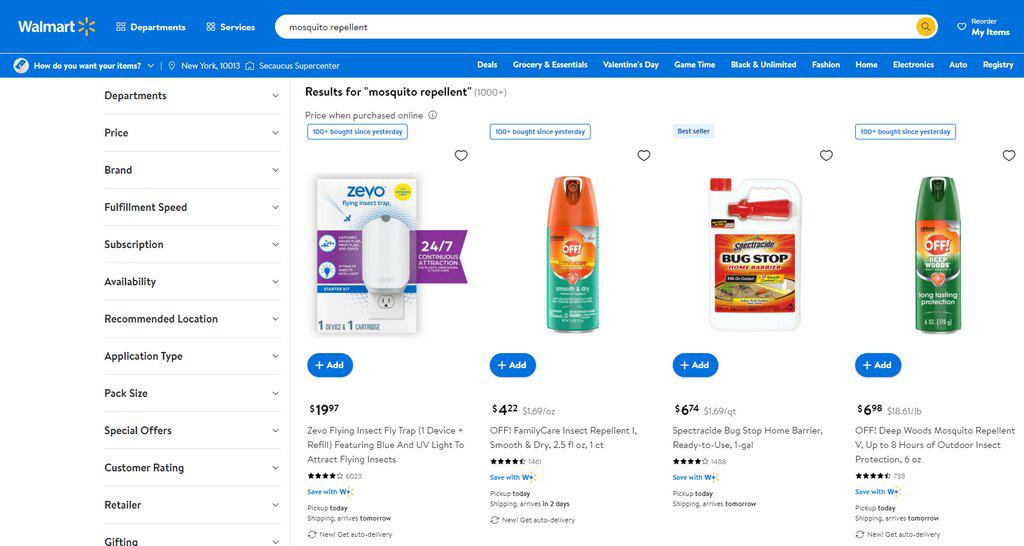In this image, we see a detailed webpage of Walmart. The top navigation bar prominently features various categories such as Departments, Price, Brand, Fulfillment Speed, Availability, Recommended Location, Application Type, Pack Size, Special Offers, Customer Rating, Retailer, and Gift Options.

The search bar contains the text "Mosquito Repellent" indicating a specific search query. Additionally, there are sections titled "How Do You Want Your Items," "New York," "10013," and "Circus Supercenter," suggesting location-specific shopping options.

Further down the page, a plethora of other categories are visible, including Deals, Grocery & Essentials, Valentine's Day, Game Time, Black & Unlimited, Fashion, Home, Electronics, Auto, Registry, and options to Reorder My Items.

There’s a highlighted product feature that shows "Price when purchased online: $6.74," for the product "Zevo Flying Insect Trap." A tagline mentions "100+ bought since yesterday," indicating its popularity. Other related items like "Spectra Seed," "Box Stop," and "Home Barrier" are also mentioned. The detailed choices denote a comprehensive shopping experience tailored for user convenience.